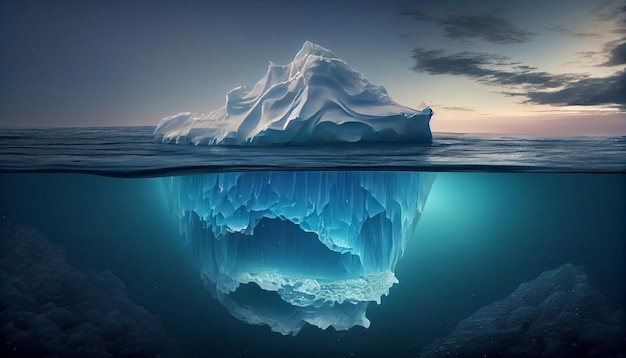The image depicts an exquisitely detailed, digitally created iceberg scene with an emphasis on both above and below the waterline. At the forefront, a large, v-shaped iceberg dominates the still, mirror-like water, its surface revealing a perfect reflection with no visible ripples to disturb the tranquility. Above the waterline, the iceberg presents a striking white with hints of blue shading, resembling a mountain of ice. The sky forms a dramatic background, featuring a gradient of evening hues from dark blue on the left to lighter shades with subtle yellow and pink tints on the right, suggesting a setting sun, accompanied by sparse clouds. Below the water’s surface, the scene is equally illuminated, showcasing the submerged part of the iceberg which expands into a semicircular shape. The turquoise-blue water is crystal clear, allowing a glimpse of underwater glaciers and rocks. The overall image is horizontal and rectangular, capturing the serene and pristine beauty of the glacial landscape.